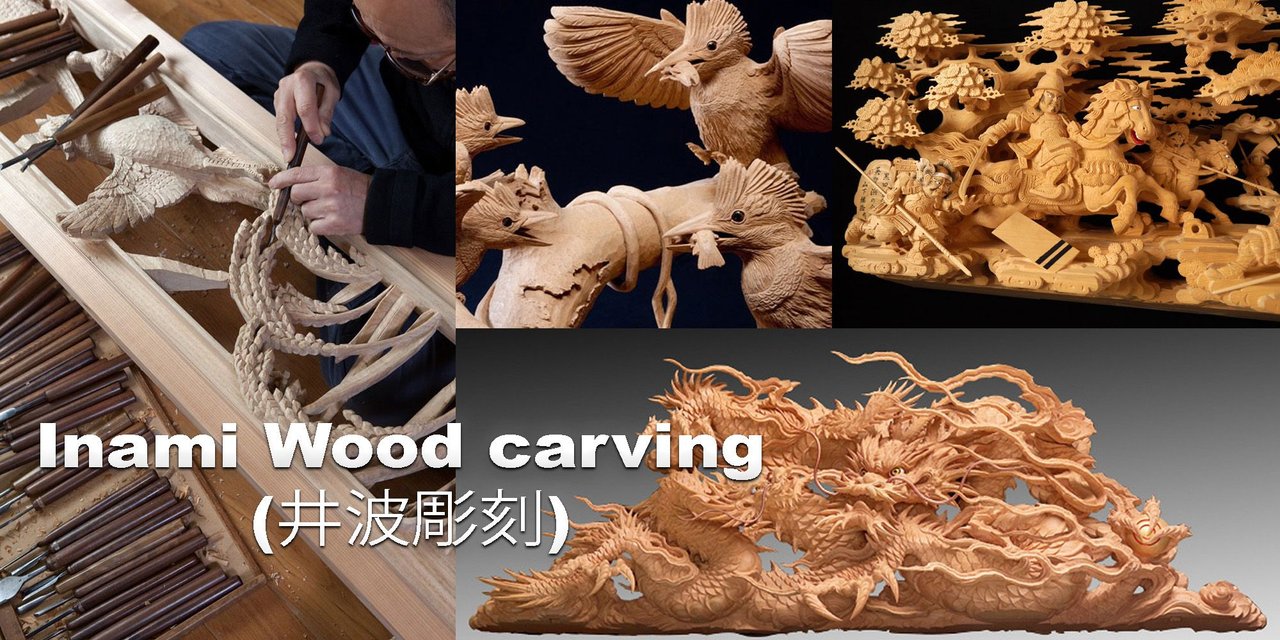The image is an elaborate collage showcasing Inami wood carving. The central focus is on a man, featured in a long left-side photograph, who is meticulously hand-carving a wooden panel. He is dressed in long-sleeve black clothing and blue trousers and wears glasses. The man is seated on the ground, working on a piece of light-colored, untreated wood, depicting what seems to be a bird and leaves. Surrounding him are various smaller carving tools laid out on the wood.

In the middle of the collage, bold sans-serif text reads "Inami Woodcarving," accompanied by four Chinese characters in parentheses, presumably translating the phrase. On the right side of the image are three distinct framed wood carvings, each showcasing different scenes. The first frame features birds holding prey, the second displays people on horses, and the third presents intricate dragon designs. These carvings are stained in rich colors like light brown, gold, and beige, highlighting their elaborate details.